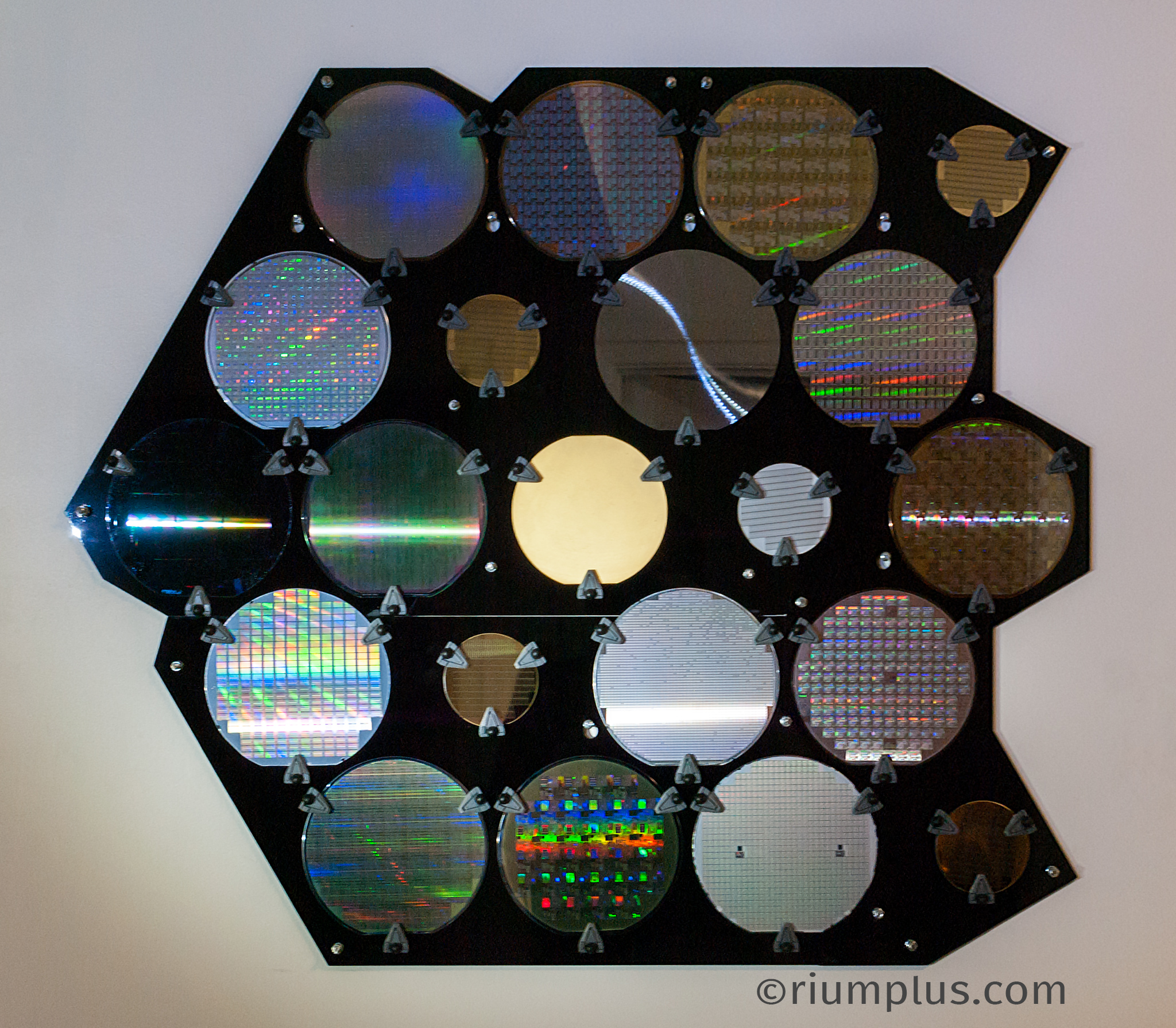The image captures a striking art piece mounted on a wall with a dual-tone background—beige at the bottom and grayish at the top. The piece itself is an angular, geometric structure resembling a stylized fish, crafted from black plastic. It features multiple round, mirror-like silicon wafers affixed with triangular pins. These wafers, resembling CDs without central holes, exhibit various colorful patterns and reflective surfaces. Some wafers shine with rainbow hues, while others have blotches of bright colors or silver with grayish lines. The wafers’ reflective properties suggest a detailed craftsmanship akin to microconductors, hinting at a complex interplay of light. The artwork merges modern aesthetics with technological elements, dynamically exploring light and color reflections. The bottom of the piece is marked with the inscription "ryanplus.com."